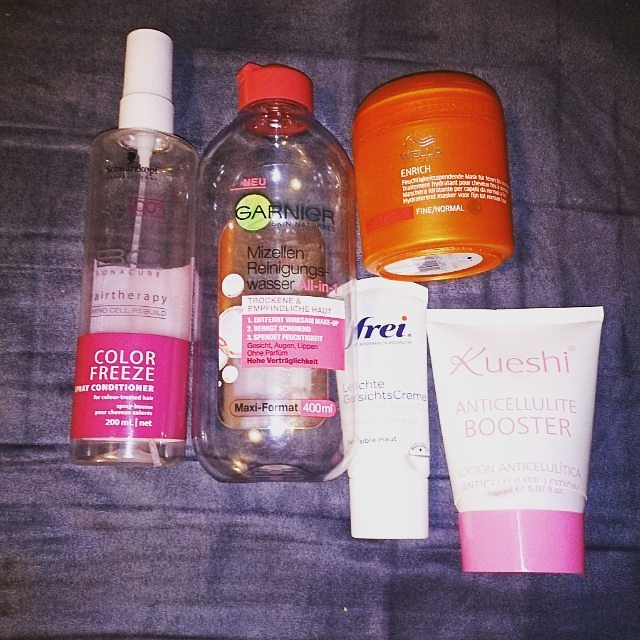The image features a carefully arranged collection of five beauty products resting on a gray, polished fabric background. Starting from the left, the first item is a spray bottle with a white cap designed in pink and white, labeled "Color Freeze Conditioner" in white text against the pink background. Next to it, a transparent bottle with a red cap showcases the brand name "Garnier" in black letters on a round green background. The third product is a white tube labeled "frei," spelled F-R-E-I. To its right, there is a squeeze cap bottle with a pink cap and pink text on a white body, which reads "Anti-Cellulite Booster." Lastly, the collection includes an orange container marked with the words "Wella" and "Rich."